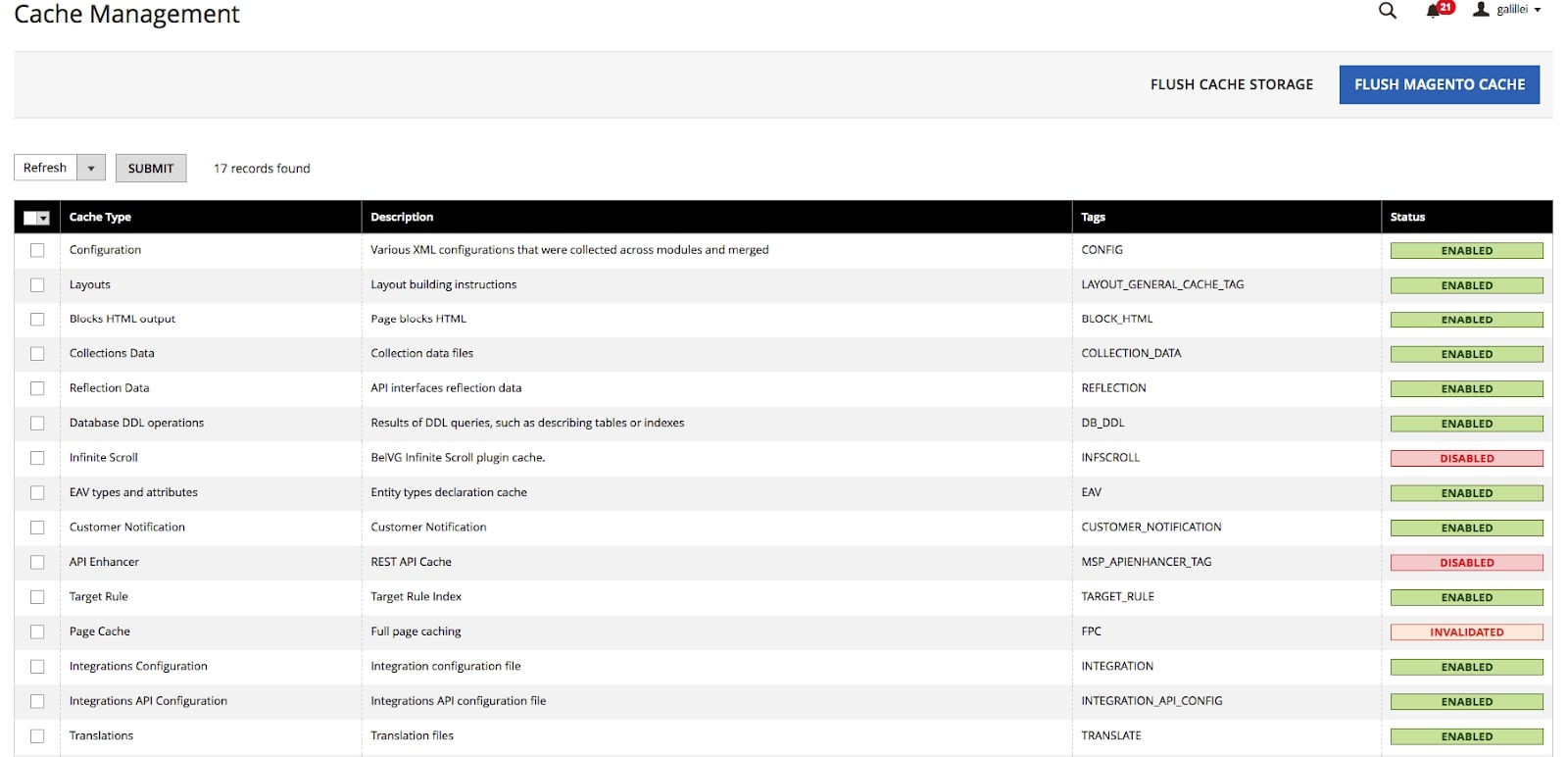This is a detailed screenshot of a webpage displaying the Cache Management section. In the top left corner, the text "Cache Management" is prominently displayed in black. To its right, a search bar is visible, followed by alert notifications and a login username. Below this, a gray banner runs horizontally, with the text "Flush Cache Storage" in small black letters situated to the right. Adjacent to this text is a blue button labeled "Flush Magento Cache."

Underneath the gray banner, the webpage features a white background. On the left-hand side, there is a drop-down box currently set to "Refresh," accompanied by a gray submit button. To the right of this button, the page indicates that "17 records" have been found. Below this information, a black horizontal bar spans the width of the page, delineating categories listed as "Cache Storage," "Description," "Tags," and "Status." In the top left corner of this black bar, there is a drop-down box allowing users to select or deselect all entries.